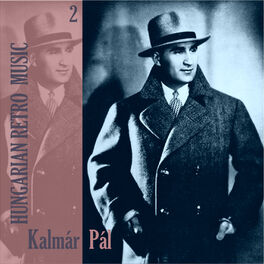The image features a black-and-white photo of a smartly dressed man wearing a white shirt with a two-tone tie, a double-breasted black wool coat with a large collar, and a white hat adorned with a black ribbon around its circumference. The man is gazing off to the right with his hands in his pockets. The background is predominantly white with some black elements. To the left of the main image, a section tinted in pinkish-purple showcases the same photograph, creating a duplicated effect. This left portion also includes black text that reads "Kalmar Pal" at the bottom and "Hungarian Retro Music" vertically. The pink-tinted segment additionally features a number two at the top.